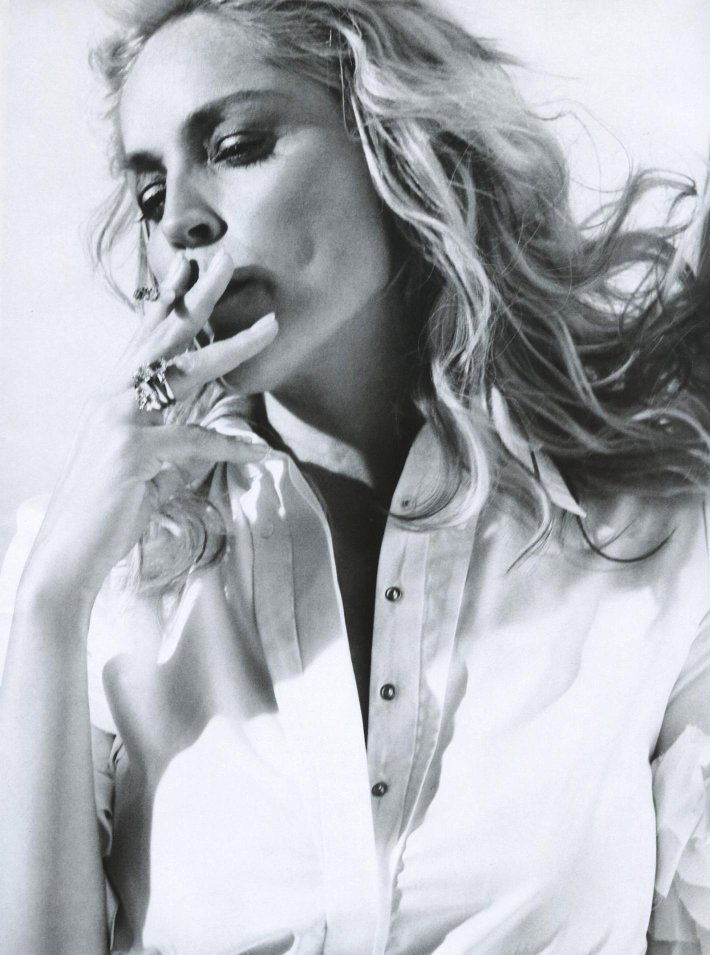This vertical black-and-white photograph features a young woman with long, wavy, blonde hair cascading past her shoulders. Her delicate features are highlighted by the contrast in the image. She is wearing an almost fully unbuttoned white blouse with long sleeves, accentuated by silver-colored buttons. Her right hand is raised to her mouth, partially obscuring her lips, and she appears to be holding a cigarette between her fingers, which are adorned with multiple rings. Her eyes are half-closed, suggesting she is savoring the moment or lost in thought. She is facing the camera but looking slightly downward and to her right. The background is a plain white or light gray, which further emphasizes her figure. The overall composition, with prominent shadows and her tousled hair, gives an impression of relaxed elegance.